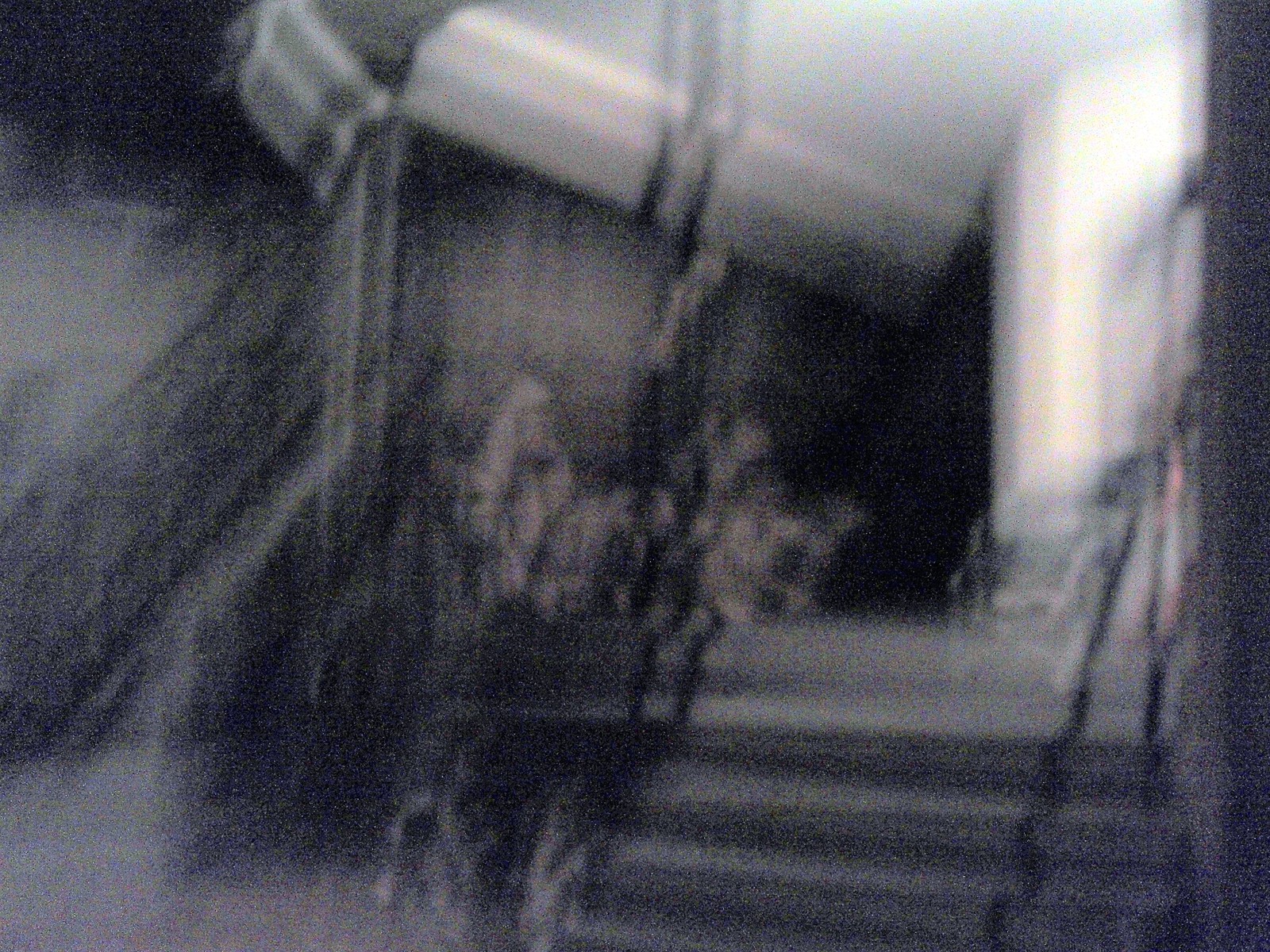This black and white photograph depicts the front facade of a house with a slightly blurred appearance. The exterior of the house has a gray tone, complemented by a prominent, large window adorned with delicate, white sheer curtains. Just in front of the window sits a part of a chair, hinting at a sitting area, and lush plants add a touch of greenery to the scene. The front porch is defined by black iron railings, which lead up to it via roughly four concrete steps. Surrounding the porch are additional plants that bring life to the entrance. Encircling the property is a solid concrete fence, adorned with subtle shadowing that adds depth to the image.